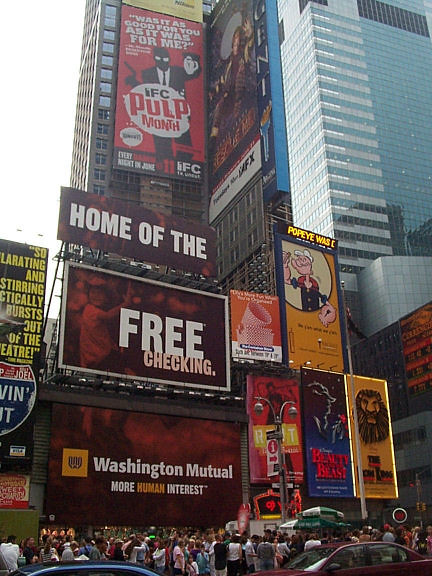This image showcases a bustling cityscape, dominated by an exceptionally tall building that spans the entire height of the frame, appearing to have at least 100 stories. Near the bottom of the scene, two cars are visible: a blue car on the left and a purplish-red car on the right. Positioned behind these vehicles is a crowd of people, captured from the back, adding a sense of urban activity. 

The building is adorned with various signs. At the base, a square sign for "Washington Mutual" with the phrase "More Human Interest" is noticeable. Directly above, another sign promotes "Free Checking" with a red background and white square. Ascending further, a red-background sign features the text "Home of the" in white letters. Higher up is an advertisement for "KFC Palt Month," also displayed on a red background with red, white, and black text.

To the right at street level, the distinctive orange sign of Popeye's stands out, featuring a circular cutout. Below this are three additional signs likely related to movies, hinting at a nearby theater or entertainment district.

In the top left corner of the image, the sky peeks through, contrasting with the imposing vertical structure of the building. The overall scene is a vivid representation of urban life and commercial signage, set against the backdrop of an impressive skyscraper.